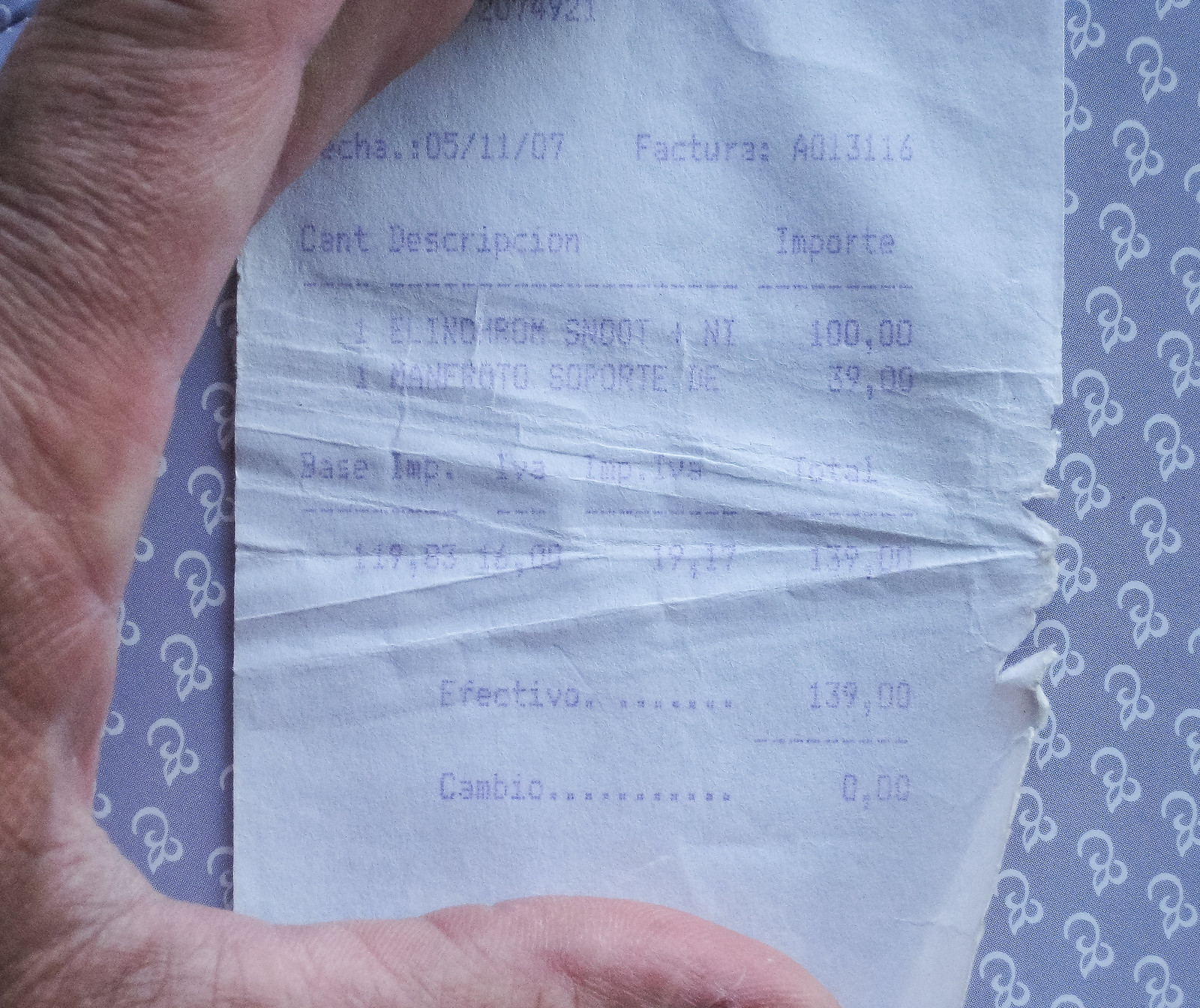A close-up image features a slightly worn receipt held open by a man's left hand. The receipt, printed on white paper with blue ink, is dated May 11, 2007. It is not in English but in Spanish, with notable words like "fractura" and specific numbers visible. The description includes an item count and an impressive total, appearing to be significant, with “import” and “100,000” mentioned in relation to some category of elder arms or similar, hinting at a large transaction. The total amount listed is “139” followed by an unspecified amount. The background consists of a blue tablecloth or wallpaper, decorated with white squiggle patterns, adding a layer of texture to the scene. The overall impression is that of an old receipt, preserved with some signs of handling and age.